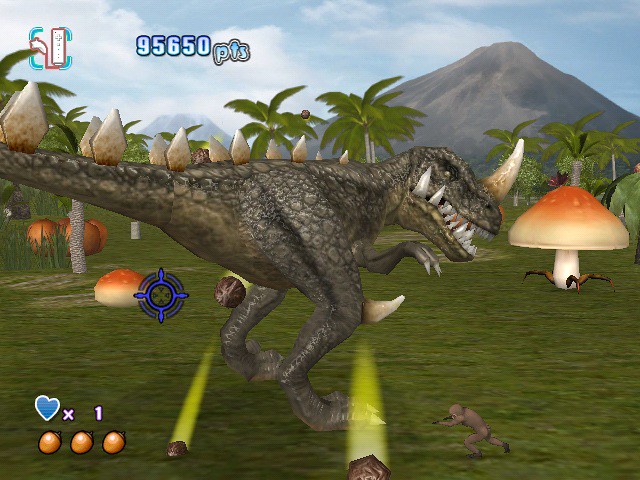In this vibrant and action-packed video game scene, a small, armed character stands courageously in front of a colossal, hybrid dinosaur. The creature, reminiscent of a T-Rex with its massive teeth and formidable presence, possesses unique features such as a prominent horn protruding from its head and another unusual horn jutting out from its knee area. The dinosaur's back is adorned with spiky plates akin to a Stegosaurus, emphasizing its chimeric nature. The backdrop features a mountainous terrain dotted with palm trees, adding a tropical feel to the environment. Scattered throughout the background, mushrooms add a whimsical touch. In the lower left corner of the screen, three acorns and a blue heart icon labeled "×1" are visible, indicating possible game collectibles or resources. Ambient lights cast a glow both in front of and behind the dinosaur, enhancing the dramatic confrontation.